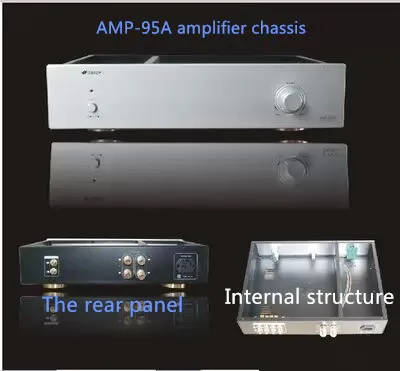The image appears to be a detailed screen grab, possibly from a service manual, showcasing the AMP-95A Amplifier Chassis against a black background. At the top of the image, "AMP-95A" is prominently displayed in blue capital letters, followed by "amplifier chassis" in lowercase. The image is divided into three sections: 

1. The upper section displays the front view of a silver amplifier with an on/off push button on the left and a volume knob on the right. This device is reflecting on the surface it sits on, creating a mirror image effect, making it appear as if there are two stacked units.

2. The lower left section, labeled "Rear Panel" in blue text, shows the back view of the amplifier, featuring various input and output connectors, although the specifics of these connectors are not clearly visible.

3. The lower right section, labeled "Internal Structure" in white text, depicts the amplifier's internals, focusing on the empty chassis setup without its electronic components. 

The image uses various shades of gray, black, light blue, off-black, and white, along with a touch of green. The layout seems to cater to individuals looking to understand or repair the amplifier, highlighting essential parts and structure for educational or purchasing purposes.